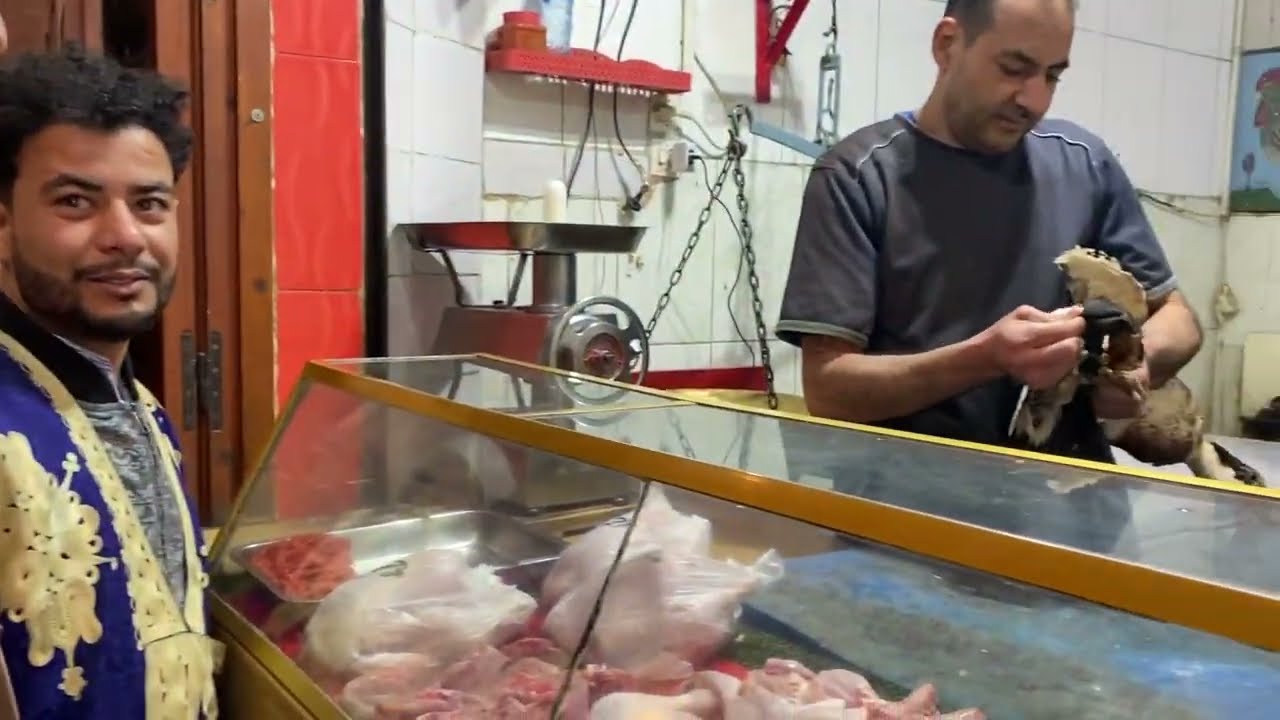In this detailed image, we see the inside of a bustling meat shop, possibly set in a location such as Mexico or the Middle East. Dominating the scene is a glass display case with brass trim showcasing an array of meats, including whole chickens, chicken feet, and ground meat. The meats are visually distinct within the glass case, some packaged in bags.

Behind the counter stands a butcher in a gray t-shirt with thinning hair at the front and a black, five o'clock shadow beard. His attention is focused downward as he tends to a piece of meat, possibly a duck or some other type of animal, adding a sense of purpose to his actions. Closer to the camera, on the left side of the frame, is a customer with thick, black hair and a full beard, dressed in a blue vest adorned with white designs over a gray shirt.

The background is split into two distinct areas: a white tiled wall with a mounted, hand-operated meat grinder attached via a chain, and farther back, the wall transitions to red tiles around what appears to be a meat locker door. Additional details include a red shelf holding a jar with a red lid, adding to the shop's character.

Overall, the image captures a candid moment in the daily operations of a small meat market with intricate details that highlight the setting and attire of the individuals within it.